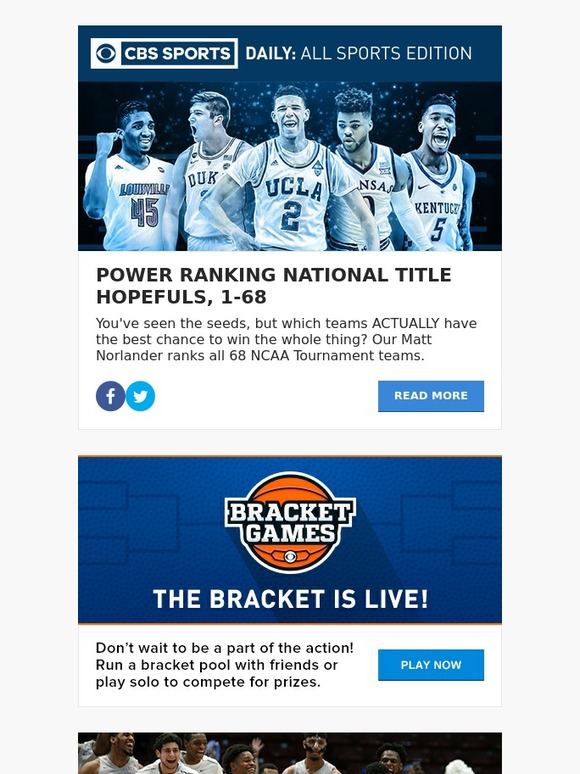CBS Sports Daily presents the All-Sport Edition featuring NBA Power Rankings. The cover image showcases five basketball players representing prominent NCAA teams: Louisville, Duke, UCLA, Kansas, and Kentucky. Below the players, a headline reads: "Power Ranking National Title Hopefuls – One through Sixty-Eight." Matt Norlander ranks all 68 NCAA Tournament teams, highlighting those with the highest chances of winning the championship. A blue button invites readers to "Read More," and social media icons for Facebook and Twitter facilitate sharing. 

Beneath this, a black banner featuring an orange basketball promotes "Bracket Games," encouraging readers to participate in bracket pools with friends or individually for a chance to win prizes. The background predominantly features white, accented with various shades of blue, black, and orange elements. The lower section of the image displays a photograph, partially cropped, showing the heads of six individuals of diverse backgrounds. The overall design combines sporty aesthetics with engaging content, promising in-depth analysis and interactive viewer participation.